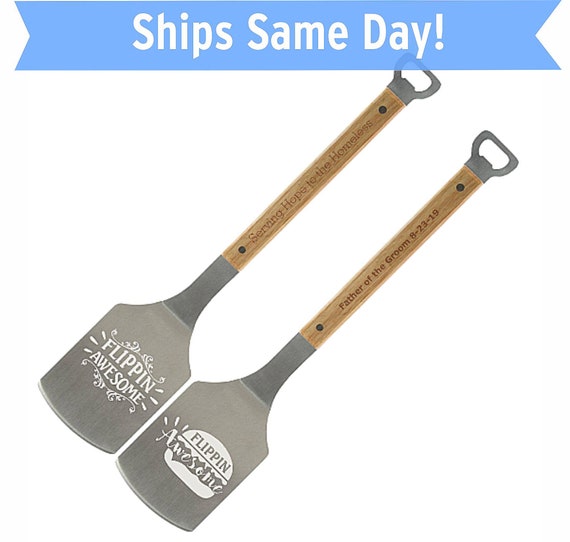The image is an advertisement showcasing two spatula flippers. At the top of the image is a medium blue, periwinkle-colored banner with white text that reads, "Ships Same Day!" Below the banner are the two spatulas, each featuring distinctive designs and inscriptions.

The spatulas have wooden handles and gray metal spatula heads, shaped like squares rounded at the bottom. The first spatula displays the phrase "Flippin' Awesome" in word art on the spatula head, with "Serving Hope to the Homeless" engraved on the handle. The second spatula also bears the phrase "Flippin' Awesome," but in a design shaped like a burger, with the word "Awesome" inside the burger image. Its handle is inscribed with "Father of the Groom, 6-23-19." Both spatulas have hooks at the top of their handles for convenient storage.